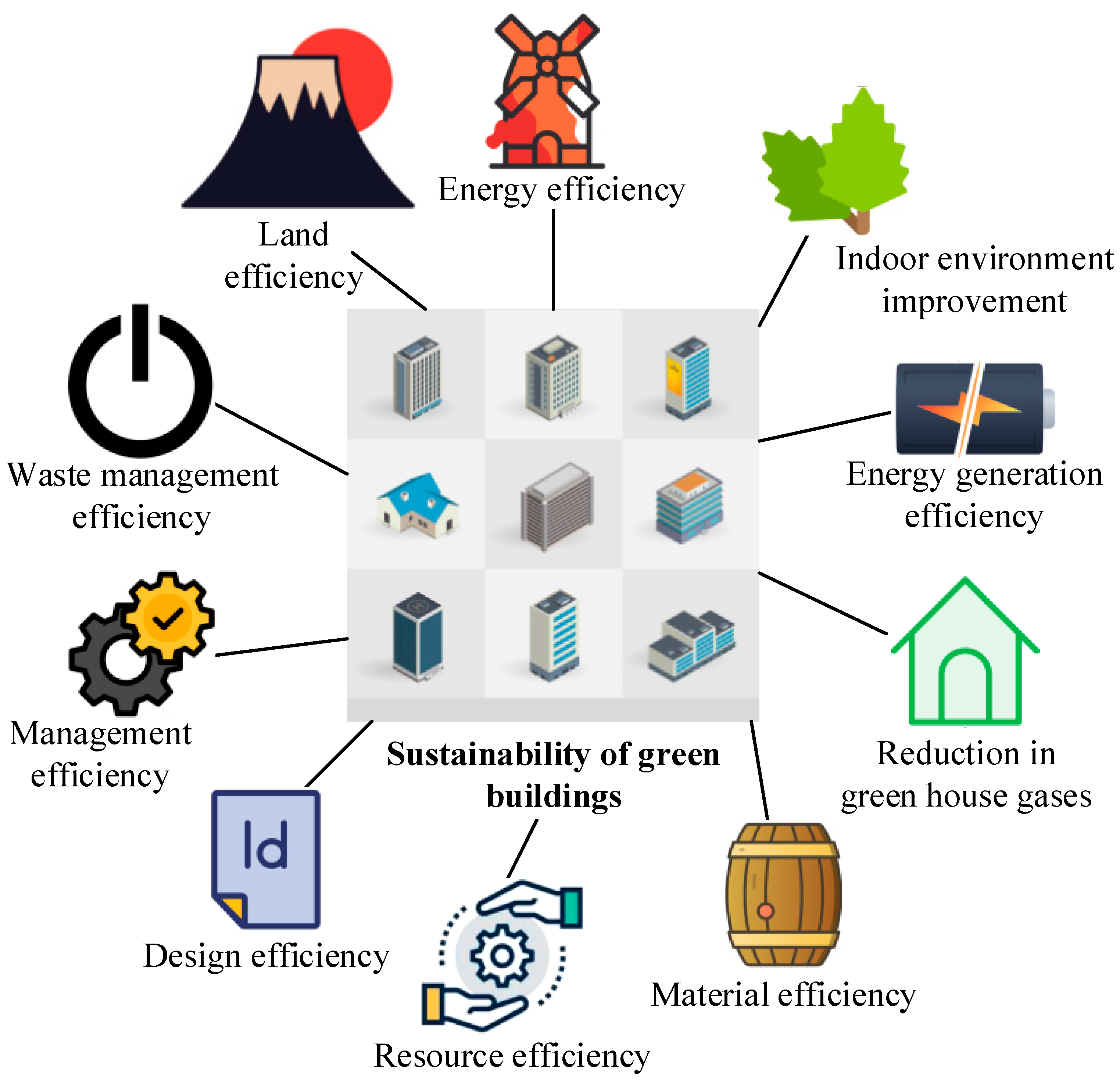This diagram illustrates the sustainability aspects of green buildings through a central grid of nine alternating light and dark gray blocks, each depicting a building type, such as skyscrapers, houses, and factories. Surrounding this grid in a circular pattern are categories that define the sustainable qualities of these buildings, each accompanied by an illustrative icon. At the top at 12 o'clock is "Energy Efficiency," marked by an orange windmill icon. Moving clockwise, "Indoor Environment Improvement" is symbolized by leaves; "Energy Generation Efficiency" features a battery with a lightning bolt; "Reduction in Greenhouse Gases" is shown with a greenhouse icon. At the 5 o’clock position, "Material Efficiency" is represented by a wooden barrel. Directly below at 6 o'clock is "Resource Efficiency," illustrated with a cogwheel encircled by hands. To its right, "Design Efficiency" has a piece of paper labeled 'ID.' Following this, "Management Efficiency" displays two overlapping cogwheels, the top one with a checkmark and colored gold. "Waste Management Efficiency" uses the classic power symbol. Lastly, at 11 o’clock, "Land Efficiency" is depicted with a tabletop mountain and a sun backdrop. Each icon visually represents various sustainability effects of green buildings, emphasizing their holistic approach to environmental responsibility.